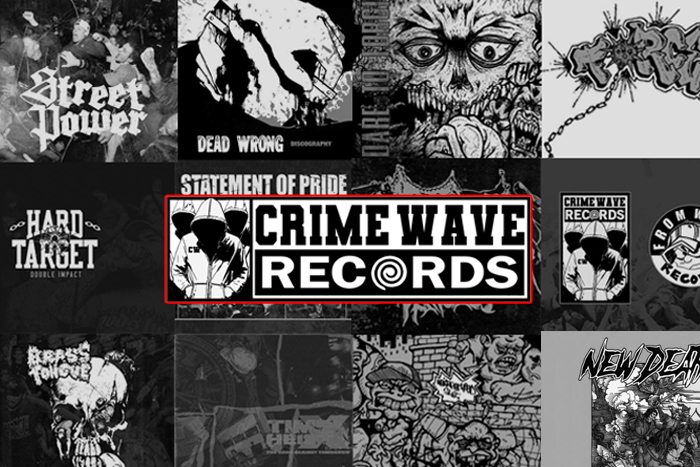This is a black-and-white advertisement for the record label Crime Wave Records, featuring images of metal or hardcore album covers. In the center, the phrase "Statement of Pride" is written in tattered text. Below it, “Crime Wave Records” is prominently displayed, surrounded by a thin red rectangle—the only color in the image aside from black, white, and gray. The O in "Records" is stylized as a whirlpool swirl, reminiscent of the hurricane emoji. Surrounding these central words are nine different album covers, with titles like "Hard Target," "Dead Wrong," "Street Power," and "New Dead." At the bottom of the image, there's a black rectangle with the word "Records" in white letters. One of the album covers features hooded figures, obscuring their faces, adding to the overall gritty and mysterious aesthetic of the advertisement.